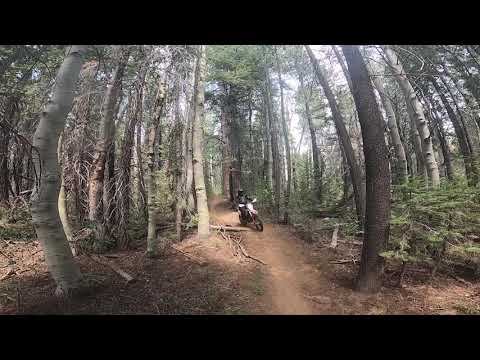The image captures a motorcyclist riding a light-colored dirt bike through a dense, dry forest. The rider, clad in a black helmet and black jacket, is navigating a muddy dirt path lined with tall, slender trees that resemble sequoias. These trees have sparse leaves predominantly at the top and some have fallen bark. The forest floor is scattered with dead twigs, fallen brush, and sparse grass, hinting at an arid environment. The path is winding, with the motorcyclist appearing to turn to the left. The blue sky with some white clouds indicates that the image was taken during daylight, with sunlight filtering through the canopy. No other animals or people are present in the scene, emphasizing the solitude of the rider as they traverse the forest.